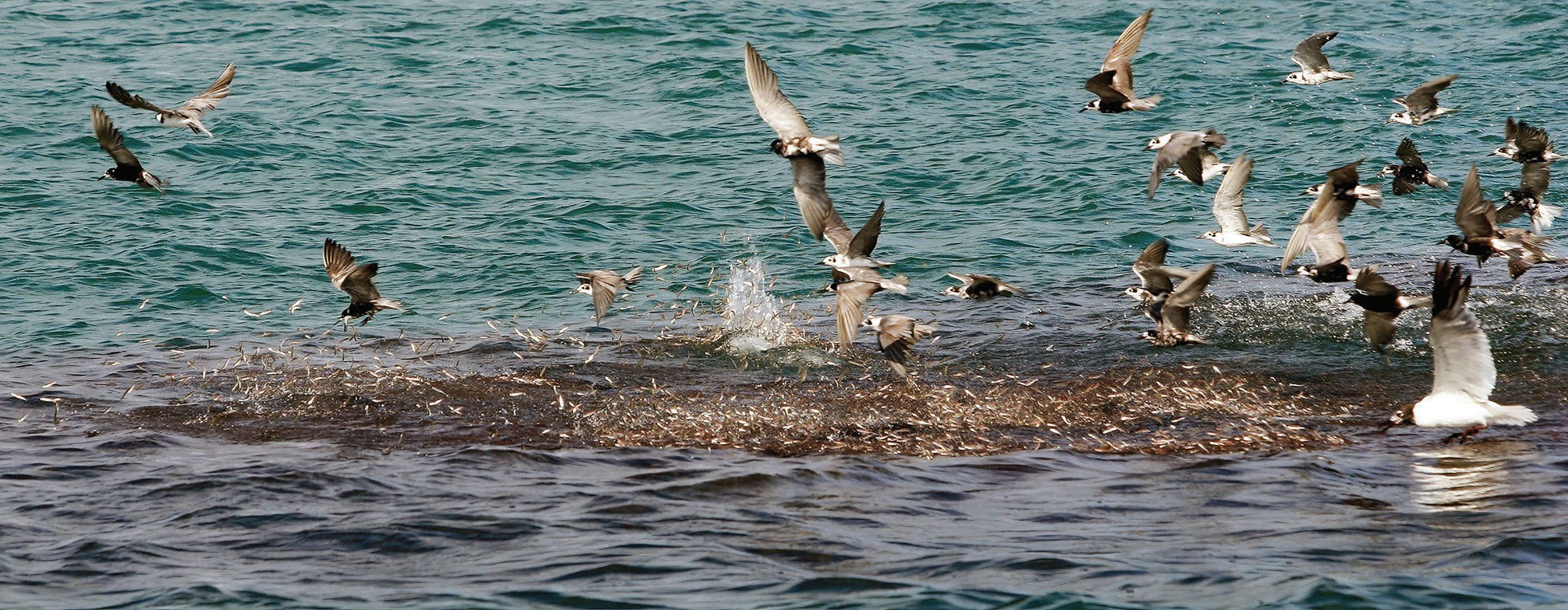This is a narrow horizontal rectangular daytime image capturing a bustling scene of seagulls amidst a choppy, multi-hued ocean. The foreground water is a dark blue, gradually lightening towards the top part of the picture. Many seagulls, identifiable by their dark heads and predominantly white bodies, are involved in frantic activity—some are perched on a narrow strip of land or rock protruding from the water, while others either sit on the surface or fly overhead. A few are mid-dive, targeting a school of small fish visible near the surface. Interestingly, within the darker patches of water, some fish even appear to be flopping above the surface. The seagulls’ wings exhibit darker edges, and some descriptions hint at brownish markings on their underbody and wingtips. The scene suggests a feeding frenzy likely induced by the presence of these small, shimmering fish or possibly bugs and plant life near the land's edge.